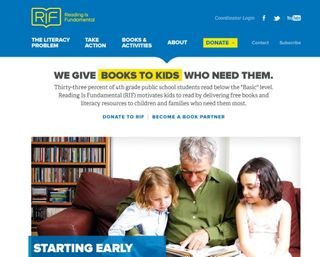This image appears to be a screenshot from a website dedicated to addressing literacy challenges among children. At the top of the webpage, enclosed in a box, are the initials "R.I.F.," representing the company's name. The navigation menu includes options labeled "The Literacy Problem," "Take Action," "Books and Activities," "About," "Donate," "Contact," and "Subscribe." There is a prominent yellow donation button featuring blue text.

The top section of the page is formatted within a blue rectangle, which functions as a header. Below this, the background transitions to white. Within this section, another blue rectangle contains the message "Starting Early" in white text.

The central message highlights the organization's mission: "We give books to kids who need them." It provides a sobering statistic that "33% of fourth grade public school students read below the basic level," affirming the critical need for their programs. The text goes on to state that Reading Is Fundamental (R.I.F.) motivates children to read by supplying free books and library resources to children and families in need.

Additionally, the image features a heartwarming photo of an older gentleman holding two young girls on his lap as they share a moment reading a book together.